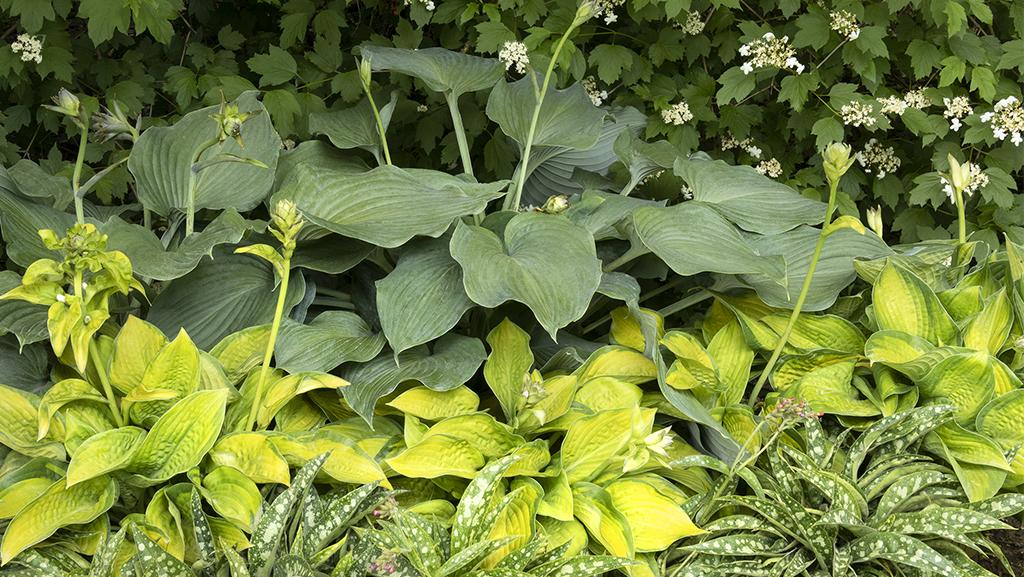This close-up photograph captures a lush, diverse garden bed teeming with various shades and types of green foliage. At the forefront, there's a plant featuring skinny, dark green leaves adorned with white speckles. Nearby, a contrasting plant displays broad, yellow-green leaves with stems shooting upward, topped by small, yet-to-bloom white flowers. Additionally, there's a plant with medium to dark green leaves that are notably larger in size. In the background, a dense bush, or possibly another type of plant with small green leaves, fills out the scene, contributing to the rich tapestry of green tones. Scattered throughout, delicate white flowers add subtle pops of brightness to the verdant landscape.